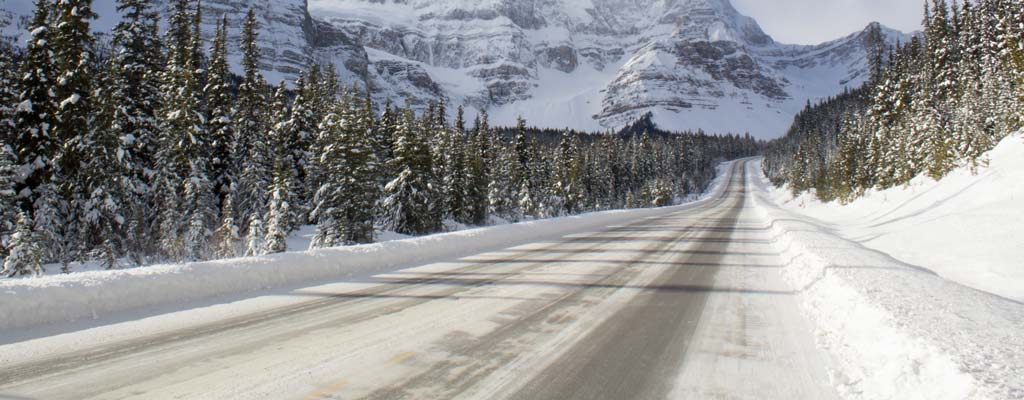In this detailed winter scene, a freshly plowed four-lane road winds through a dense forest of fir trees, with only two lanes currently usable due to the snow buildup on either side. The asphalt road, still slick with ice, features a yellow divider line peeking through the thin snow cover. Shadows from the sun-streaked evergreen trees stretch across the pavement. Lining the road, the fir trees are dusted with snow, adding to the serene winter atmosphere. In the background, a majestic, snow-covered rocky mountain bluff extends across the entire scene, its high peaks partially visible and dark brown spots hinting through the snow. The road slightly curves to the right as it leads towards the imposing mountain, creating a picturesque view. There also seems to be a distant car on the left side of the road, emphasizing the quiet, remote nature of this snowy landscape. The overall setting is that of a tranquil, yet cold, forested mountain area in the depths of winter.